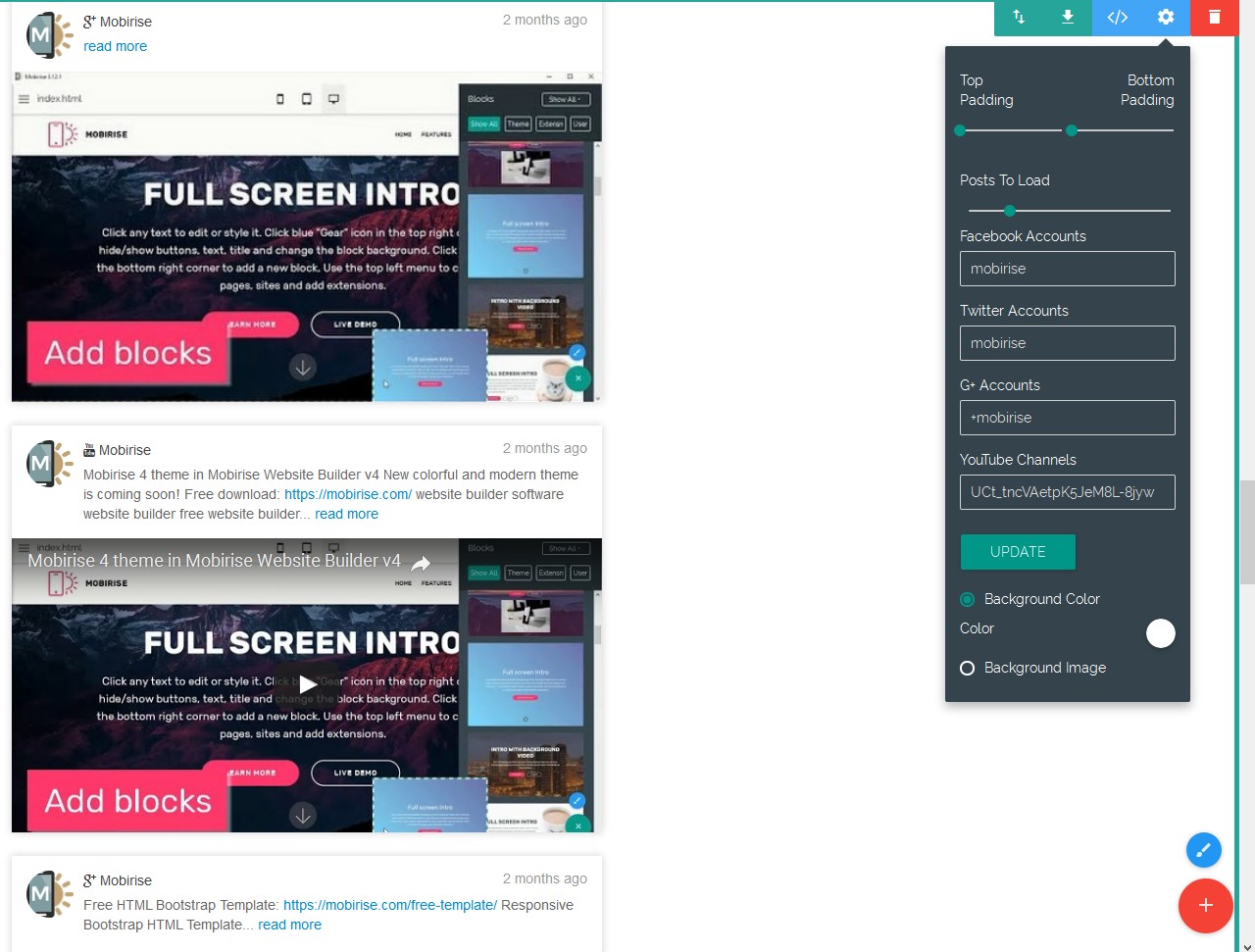This screenshot is bifurcated by a thin vertical line running through the center, creating two primary sections. 

**Right Section:** 
- A predominantly blank, white screen.
- In the upper right corner, there is a small, colorful menu.
- Adjacent to this menu, there's a larger dropdown menu emanating from a gear icon housed within a blue box.
- This dropdown menu features a dark background with white text, and includes a prominent green "Update" button.

**Left Section:** 
- This section is further subdivided into two almost identical parts, each displaying an interface with large white text that reads "Full Screen Intro."
- Both parts feature a small icon in the upper left corner next to the text "G Plus Mobilize Read More."
- At the bottom left corner of each part, there is a small red rectangle containing the text "Add Blocks."

This descriptive caption provides a clear and comprehensive overview of the visual elements present in the screenshot.